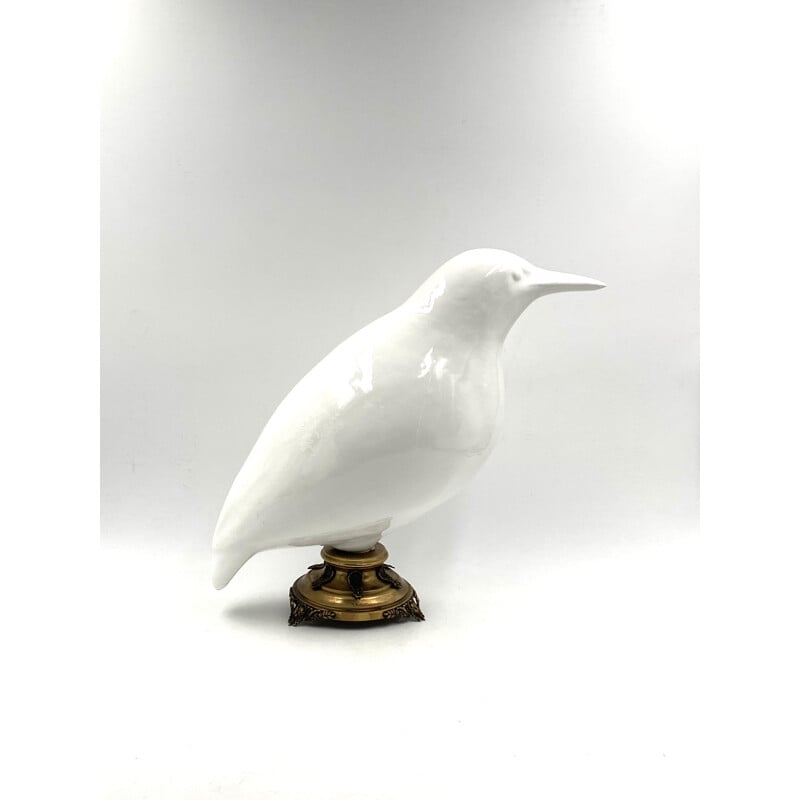The photograph features a smooth, white porcelain bird with minimal details, including a small tail pointed downward and a long, sharp beak. The bird is perched on an ornate, golden pedestal with a wide base. This pedestal includes small, darker loops extending from the base toward where the bird sits, ornate legs that connect the pedestal to the ground, and is decorated with little dots and grooves. The image is set against a white background, slightly illuminated by lights positioned at the top left and top right corners, creating a bright effect in those areas. The overall composition is clear and clean, focusing on the chubby, porcelain bird that seems to meld into the gold pedestal, reminiscent of a decorative inkwell.